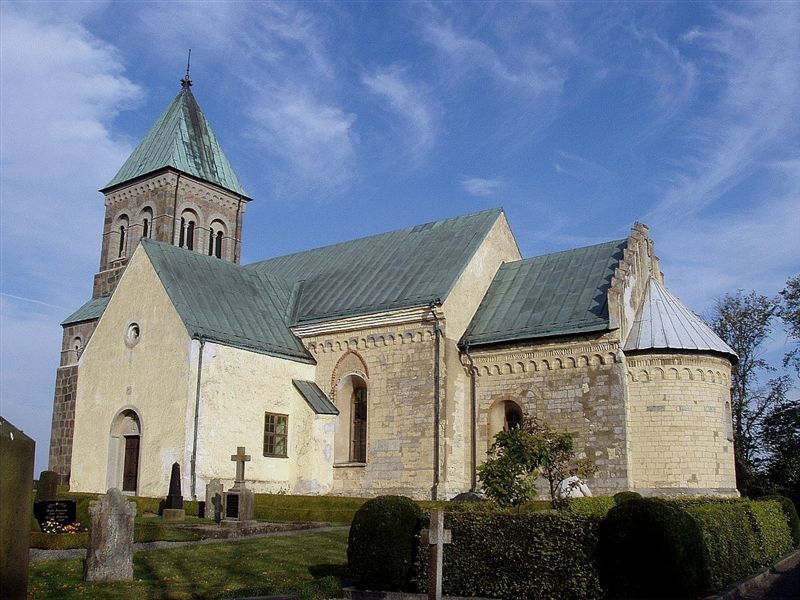The photograph showcases a historic church, predominantly filling the frame, with a bright blue sky and some clouds overhead, emphasizing its tranquil setting. The church features distinctive architecture with whitish-gray bricks and an off-white exterior, adorned with intricate brick patterns. Notably, the roofs, including a tall clock tower and a dome-shaped section, are painted green, albeit weathered and discolored in some parts. A cemetery, typical of traditional churches, sprawls to the left in the foreground, revealing several headstones, including one with a crucifix. The property is bordered on the right by well-maintained, rectangularly trimmed hedges and small bushes, adding to the preserved charm of the church. In the distance, one can also see a couple of trees, completing the serene and historical ambiance of the scene.